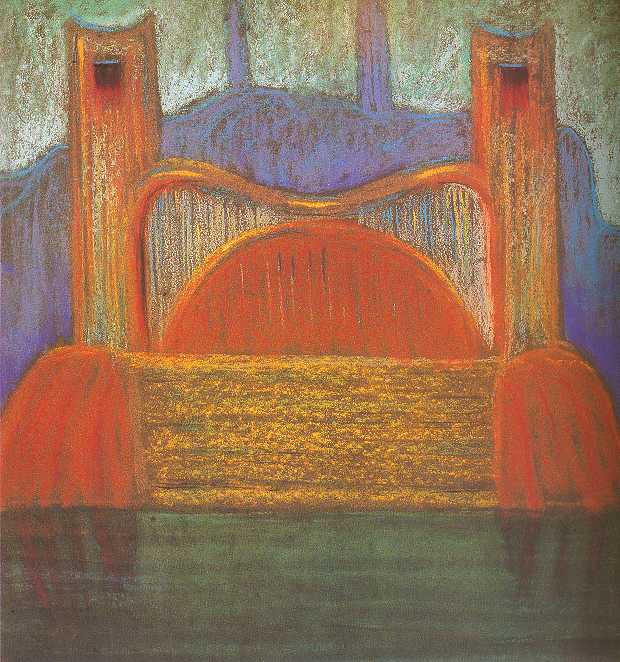The image is a richly textured and colorful pastel drawing. It depicts the foot of a bed with two tall, orange posts accented with yellow and gold details. The bed's headboard features a striking orange arch with gold highlights, adding to its visual appeal. The bed itself appears to be covered with bluish-purple linens, enhancing its vibrant appearance. Behind the bed, a purplish wall is adorned with two vertical posts. This wall gives way to an open window that allows light to pour into the scene, illuminating the composition. The floor in front of the bed is a smooth, greenish-black surface with a subtle sheen and reflections from the bedposts. The background is a mix of dark tones, highlighted with messy gray and bright purple lines, adding depth and complexity to the overall image.